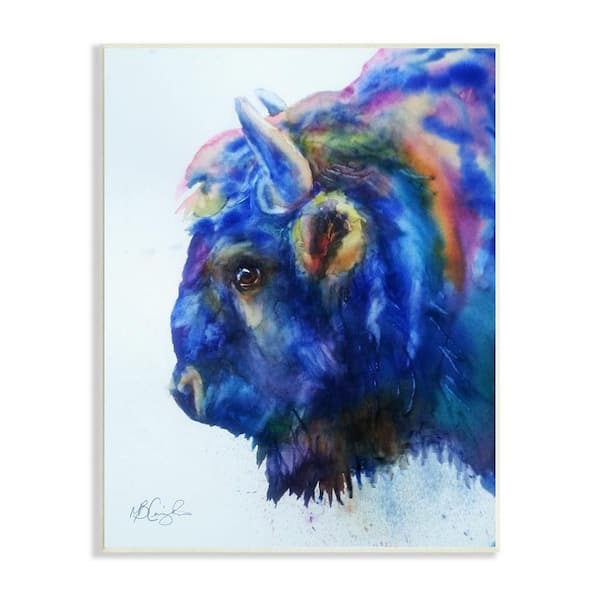This image showcases an artist's stylized painting of a young bison, prominently featuring its head and the forefront of its shoulders. Set against a light blue background, the bison is rendered in an array of vibrant colors, including various shades of blue, accented with streaks of purple, pink, orange, red, and hints of green. The animal's eye is meticulously detailed, contrasting with the softer, muted brushstrokes that define the rest of its form. The bison has medium-sized black eyes and two prominent horns extending from either side of its head, alongside a small black beard hanging from below its mouth. The bison is depicted looking sideways, offering a profile view from slightly below the neck to the front of its head. Below the image, there is an illegible signature in the lower left-hand corner, possibly identifying the artist as Pierce Street or B. Cunningham. The overall effect of the painting is one of calm and contemplation, achieved through the use of pastels and non-realistic color tones which imbue the image with a tranquil and reflective quality.